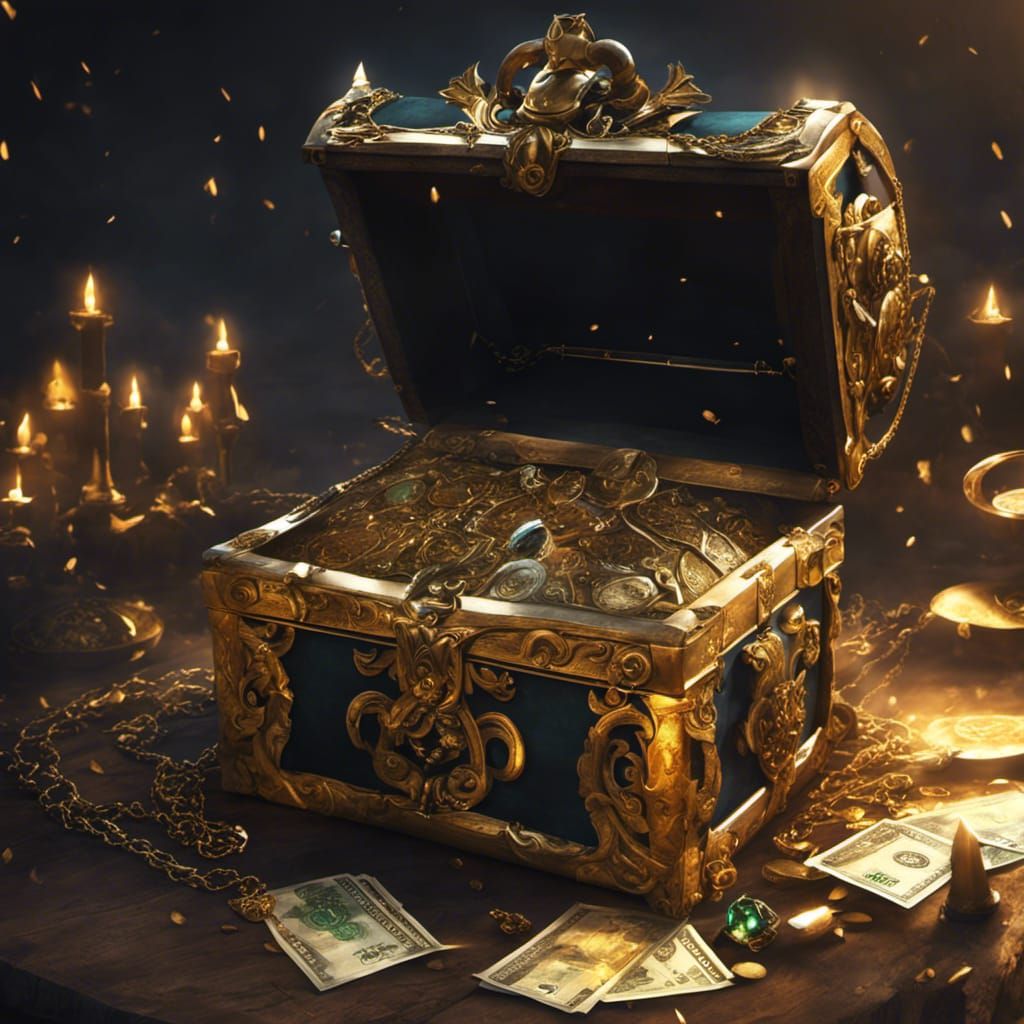The image is an AI-generated depiction of a treasure chest and various trinkets on a wooden platform, set against a black background. The centerpiece is a black chest adorned with intricate gold edging and filigree designs, partially open to reveal an abundance of gold coins inside. The top of the chest, though not fully visible, appears to be inlaid with turquoise. Surrounding the chest, the platform is cluttered with paper money of an indeterminate and unfamiliar currency, glittering jewels, gold chains, and an assortment of ornaments including brass serving plates. To the left of the treasure, a grand, multi-armed brass candelabra with numerous lit candles casts a warm glow, while a single candle stands on the right. The scene has a chaotic yet mesmerizing quality, with small tendrils of fire dancing above the scattered wealth, completing the atmospheric tableau evocative of a pirate's trove.